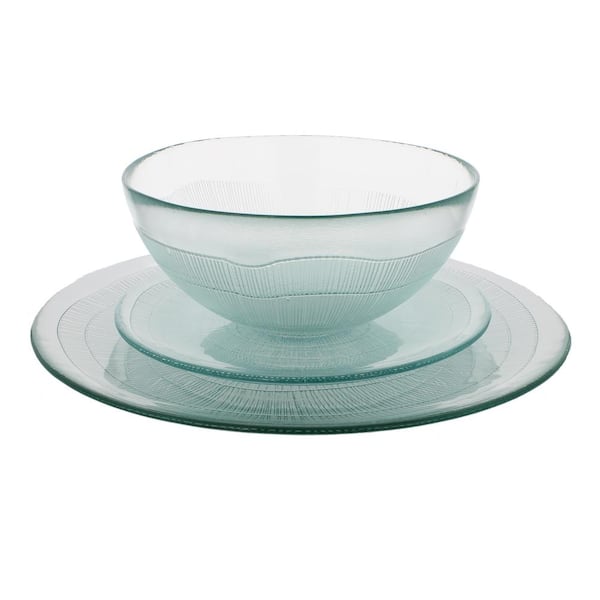This image showcases a meticulously stacked dinner set presented against a plain, white background, almost as if it's intended for a product or stock photo. At the top of the stack is a heavy-duty, clear, and opaque glass bowl with an intricate design. The bowl's rim is smooth, transitioning midway down into segmented textures resembling bands of an earthworm, with the glass giving off a light greenish-blue, ice-like hue. This reflective quality renders the glass both shiny and clean. Below the bowl is a smaller saucer, potentially a salad plate, that mirrors the same icy and glassy finish. Finally, at the bottom is a large dinner plate, characterized by its similar icy appearance and concentric circle etching that adorns its edge. The dark greenish-gray rim of the bowl and the segmented design, along with the etched lines at the center of the plates, add depth and a tactile nature to the set. The lighting, seemingly from above, enhances the clarity and sheen of the glass, making the details of the textures and colors stand out.